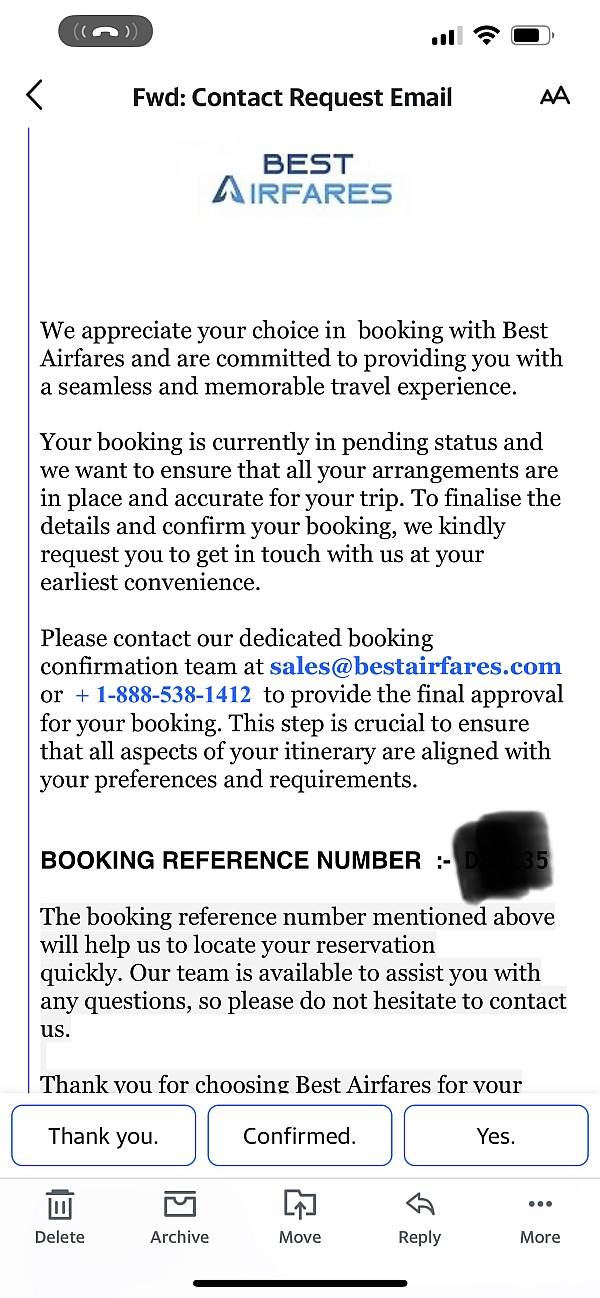**Detailed Captured Image Description:**

The image shows a forwarded contact request email from "Best Airfares." Positioned at the top of the email, the company’s logo features the words "Best Airfares," with the letter "A" stylized to resemble a tree or mountain. The message begins with an expression of gratitude: "We appreciate your choice in booking with Best Airfares and are committed to providing you with a seamless and memorable travel experience."

The email proceeds to inform the recipient that their booking is currently in a pending status and emphasizes the importance of confirming all travel arrangements. To finalize and confirm the booking, the recipient is kindly requested to reach out to Best Airfares at their earliest convenience. The email provides the contact information for the booking confirmation team, including an email address (sales@bestairfares.com) and a phone number.

The email underlines the necessity of this step to ensure that every aspect of the itinerary aligns with the recipient's preferences and requirements. It includes a "Booking Reference Number," which has been redacted with black sharpie for privacy. The email states that this reference number will help locate the reservation quickly.

Towards the end, the email assures the recipient that the team is available to assist with any questions and encourages them to contact the team without hesitation. The message signs off with a note of thanks: "Thank you for choosing Best Airfares for your," but the sentence is abruptly cut off.

This detailed description captures not only the content but also the visual elements and tone of the email, ensuring a clear and comprehensive understanding of the image.